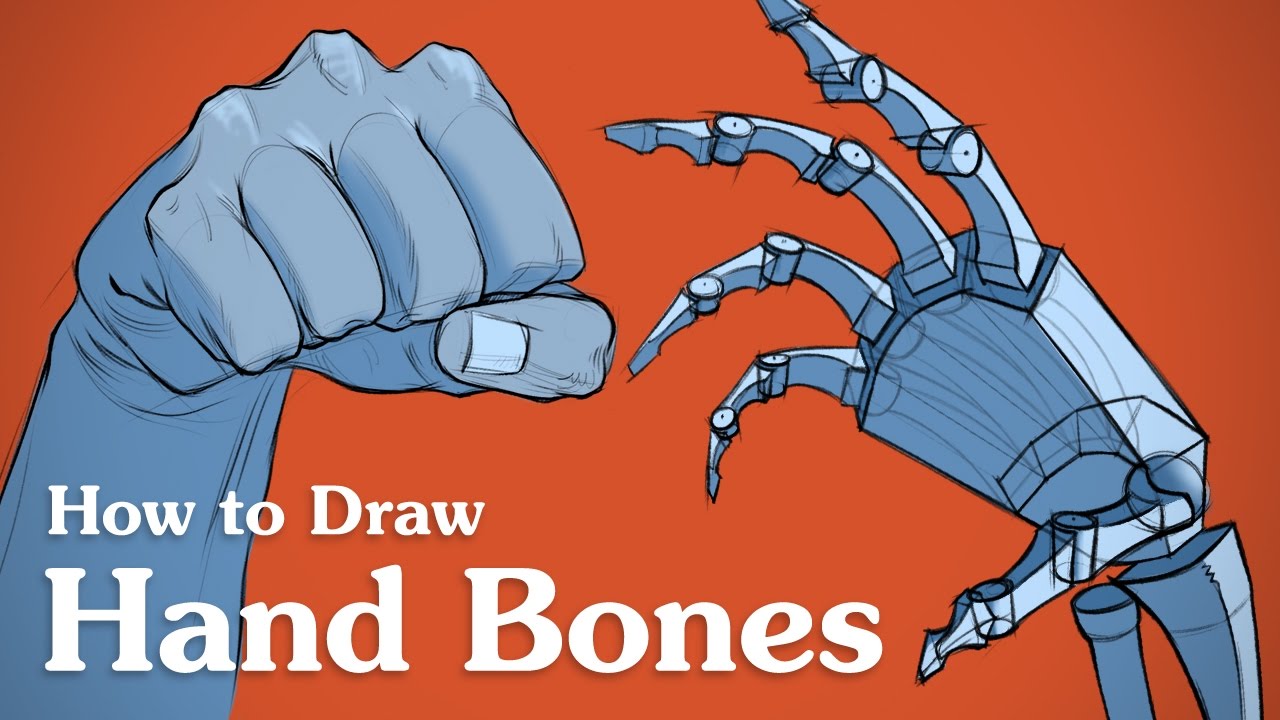The instructional image on how to draw hand bones features two detailed illustrations against a dark peach (orange) backdrop. On the left, there is a hand depicted in a clenched fist position, showcasing the thumb prominently in front. On the right, there is a drawing of a skeletal, robotic-like hand, complete with visible joints and wrist bones, and arranged as if reaching towards the clenched fist, with the fingers extended in a claw shape. Both illustrations are rendered in a gray-blue tone with sketchy lines to emphasize the technical aspects. The image is titled with "How to Draw Hand Bones" in white font at the top, with the subtitle "hand bones" placed at the bottom left.